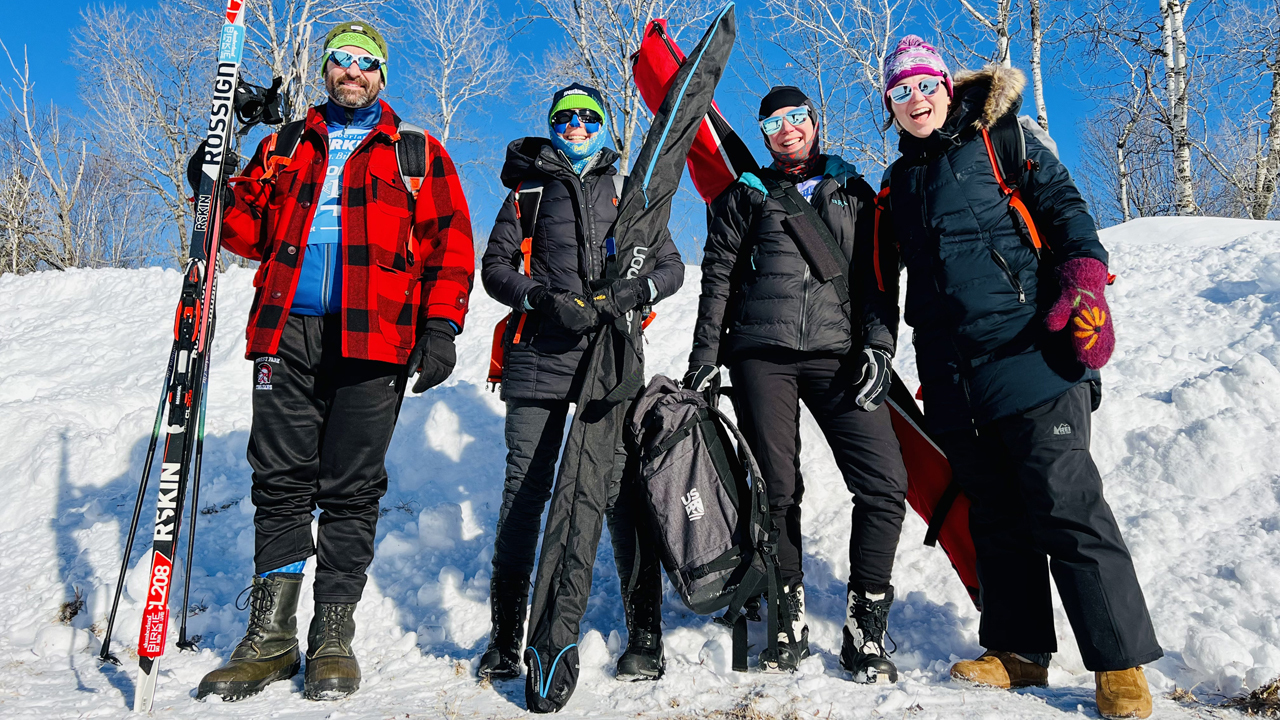In the bright sunshine of a clear blue sky day, a group of four skiers stand together against a backdrop of barren birch trees sprinkled lightly with snow. The snowy ground beneath them contrasts sharply with the vivid hues of their winter attire. 

On the far left, a man is dressed in a classic lumberjack-style red and black checkered jacket, with a blue shirt peeking from underneath. He is also wearing a knit cap, sunglasses, and green ski pants paired with black boots, and he holds his skis confidently.

Next to him, a woman is clad in black ski pants and a matching puff jacket. She accessorizes with a scarf around her head, a green cap, and sunglasses. Her skis are neatly stored in a black case she carries.

To her right, another woman stands with black pants, black puff jacket, and black boots. She has a gray tote bag and her skis hang behind her in a red case with black stripes, supported by a shoulder strap. She tops her outfit with a black hat.

On the far right, a woman dressed in a long black jacket with a fur-lined hood stands out. She pairs her outfit with black pants and beige boots. Her hands, covered in large burgundy mittens adorned with a sun motif, hint at a touch of personality. Her burgundy knit cap with a tassel and sunglasses complete her ensemble.

Together, they embody the perfect blend of functionality and style for a beautiful day on the slopes.